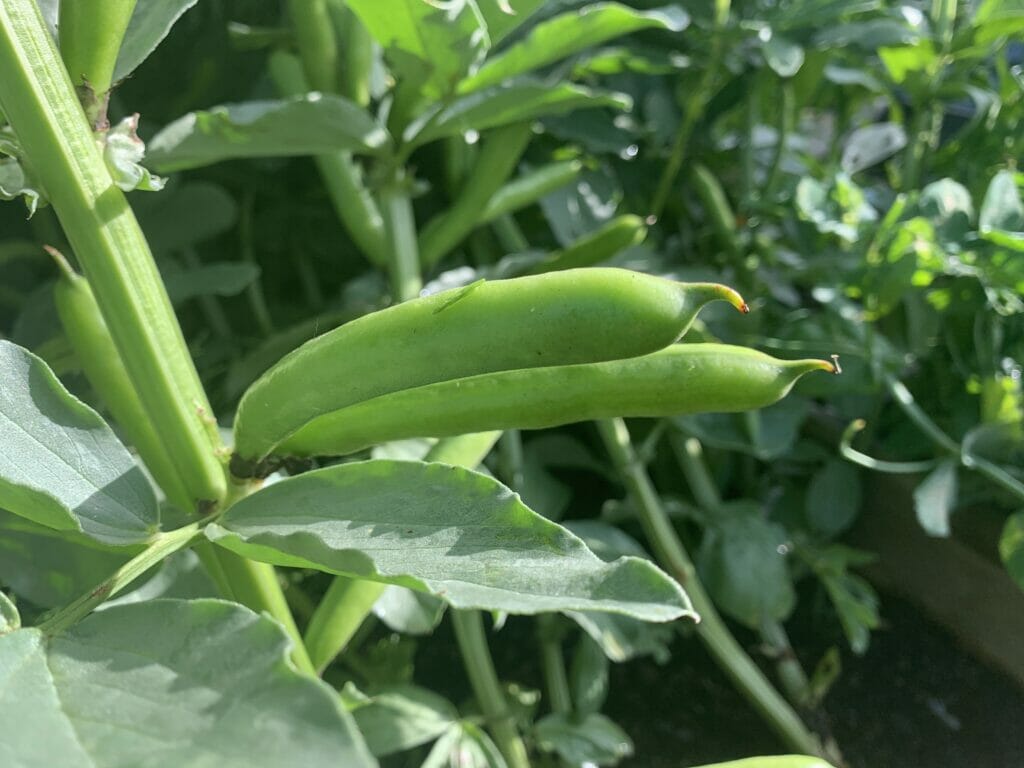In this close-up image of a garden, the focus is on a green plant with two prominent pods, resembling either snap peas or green beans, attached to its yellow-green stem. The pods are tubular and have tiny ends, with one end connected to the plant's main stem and the other tapering into a small point. The leaves in the foreground are a mottled mossy green and reflect sunlight, creating a dappled effect with shadows from the curled edges. In the background, which is softly out-of-focus, you can discern additional stems and pods along with more vibrant green foliage and shoots. The earthy garden setting is highlighted by the visible dirt, alongside the lush and varied vegetation, suggesting a well-maintained outdoor space. Overall, the image captures the lush greenery and natural sunlight of a garden scene with a variety of plant life.